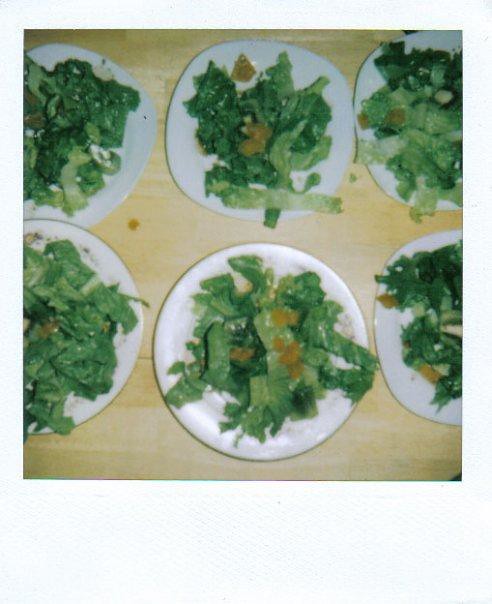This image is an overhead shot of a pale tan wooden table adorned with six plates of salad. Each plate, varying slightly in shape, is arranged with three on the top row and three on the bottom. The center plates are fully visible, while the ones on the left and right edges are partially out of frame. Four plates - the top three and the bottom-right - are rounded squares, and the bottom middle and left plates are fully round. 

The salads consist of green lettuce, possibly romaine, with little pieces of orange, which might be mandarin segments or croutons. Additionally, there are hints of cheese mirroring a Caesar salad component. The evident minimalist design of the plates and the grainy, vintage filter of the image suggest a Polaroid style, adding a nostalgic, 70s-era ambiance. A small circle of spilled dressing or sauce can be observed toward the middle-left side of the table, enhancing the casual, informal setting likely indicative of preparing for a group event, such as a dinner party or a restaurant service.